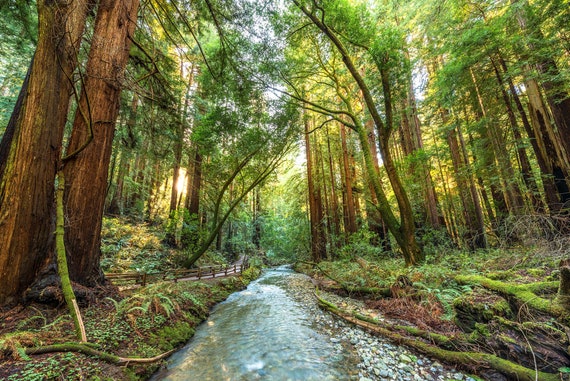The image depicts a scenic forest dominated by towering redwood trees, their rich, earthy brown bark contrasting with the dense, shadowy green of the canopy above. Sunlight dapples through the trees, creating patches of brighter green foliage amidst the shadows. In the center of the image, a crystal blue stream runs, reflecting the sky above and flanked by rocky creek beds. To the left of the stream, a small path winds its way through the ferns and shrubs, bordered by a simple rail or fence. The forest floor is dotted with fallen branches and logs, many covered in vibrant green moss. The creek, about six feet wide, meanders off into the distance, surrounded by lush greenery on either side. Above, patches of blue sky peek through the verdant canopy, further illuminating the peaceful woodland scene. The overall setting is a natural, serene forest grove, captured in vivid, realistic detail.